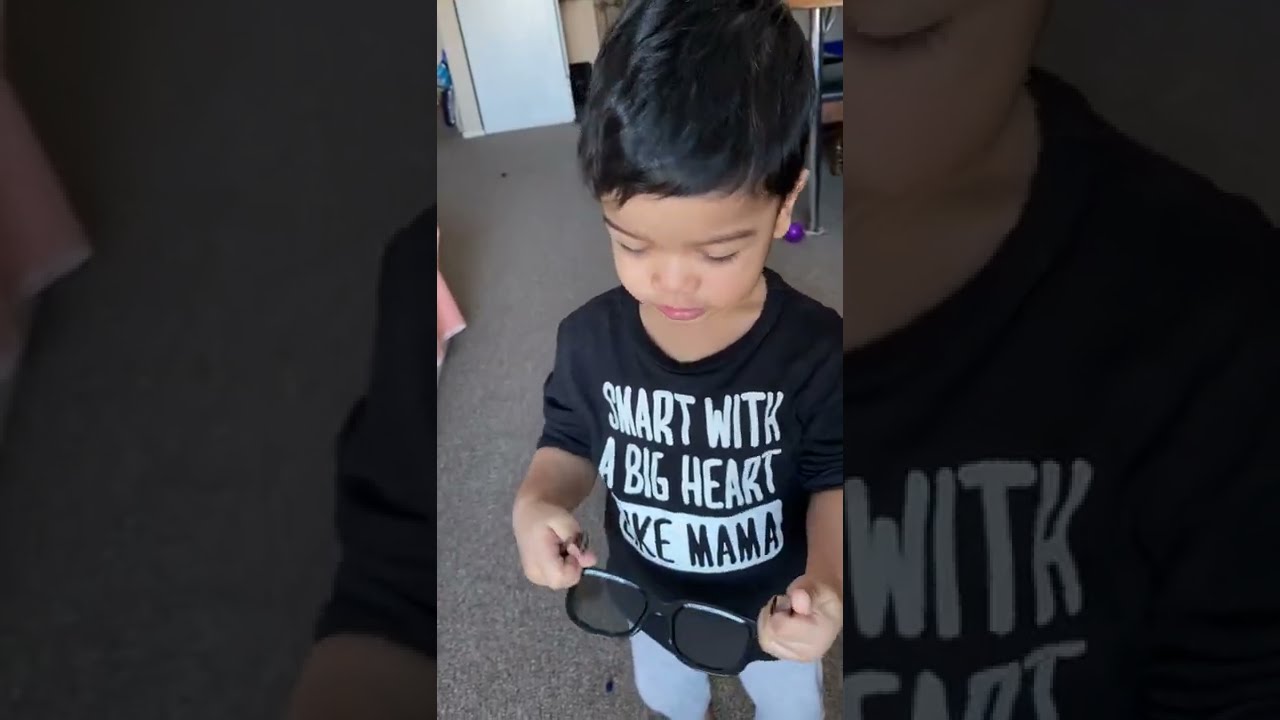This is a photograph presented as a triptych, with the left and right panels blurred and larger than the central panel. The central panel depicts a young Asian boy, possibly a toddler, standing on a low-pile gray carpet in a well-lit home setting that appears to be a living room. He has short black hair, chubby cheeks, and dark eyebrows. The boy is looking down at a pair of black sunglasses he is holding in his hands. Dressed in a black t-shirt with the white lettering "Smart with a big heart like mama," the child is also wearing blue pants. Behind him, a white wall is visible, along with a chrome metal table leg to his left, which supports an item with bits of brown, possibly a table or cart. Additionally, a purple ball is situated by his right ear near the metal leg. On the left side of the central panel, there seems to be a pink tablecloth. The left and right panels of the triptych, which are darker and blurred, contain enlarged and grayed-out elements of the main image, such as a gray floor, part of a forearm with a black sleeve, and a close-up of the boy's torso, neck, and lower face.